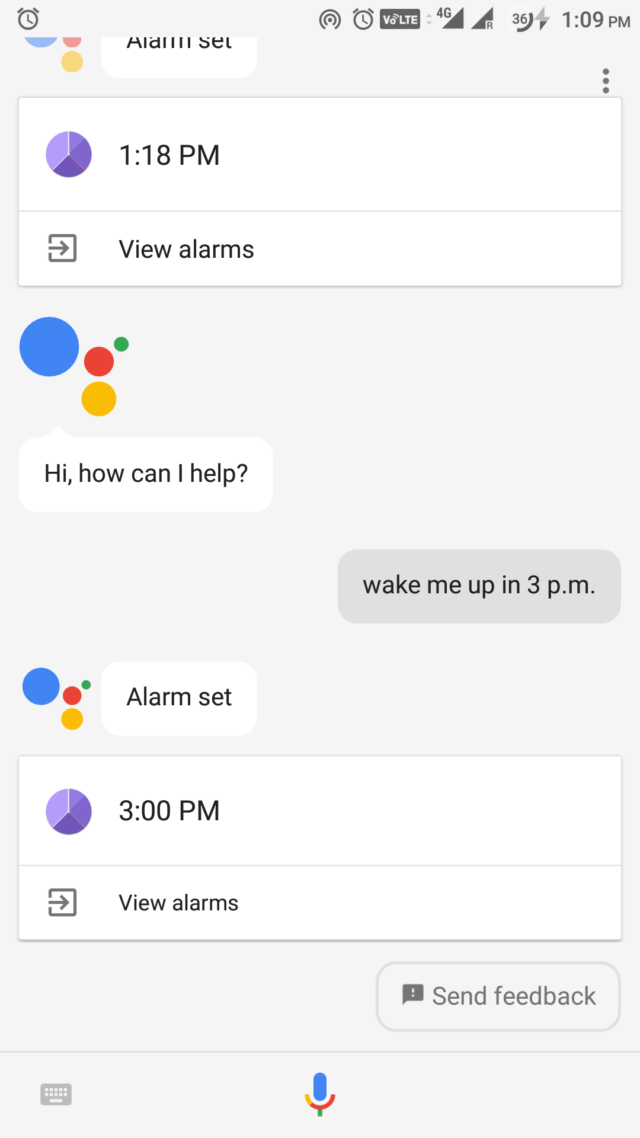A detailed caption for the image could be:

"A screenshot from a smartphone displaying a conversation interface, likely from a virtual assistant or alarm setting app. The top left corner features a clock emoji and some other symbols, while the top right shows the current time. Below these, a white box with a purple pie chart icon displays '1:18 PM' and an arrow accompanied by the text 'View Alarms'. On the left side, multicolored bubbles in blue, red, yellow, and green appear above a message bubble that reads, 'Hi, how can I help?'. To the right, a gray message bubble contains the reply, 'Wake me up at 3 PM'. Further below, another set of colorful bubbles is followed by the confirmation message, 'Alarm Set,' and another purple pie chart icon stating '3 PM' with a right-facing arrow labeled 'View Alarms'. At the bottom right corner, an oval button with the text 'Send Feedback' is visible. The very bottom of the screenshot shows a microphone icon, indicating that the user might be using voice commands to interact with the app."